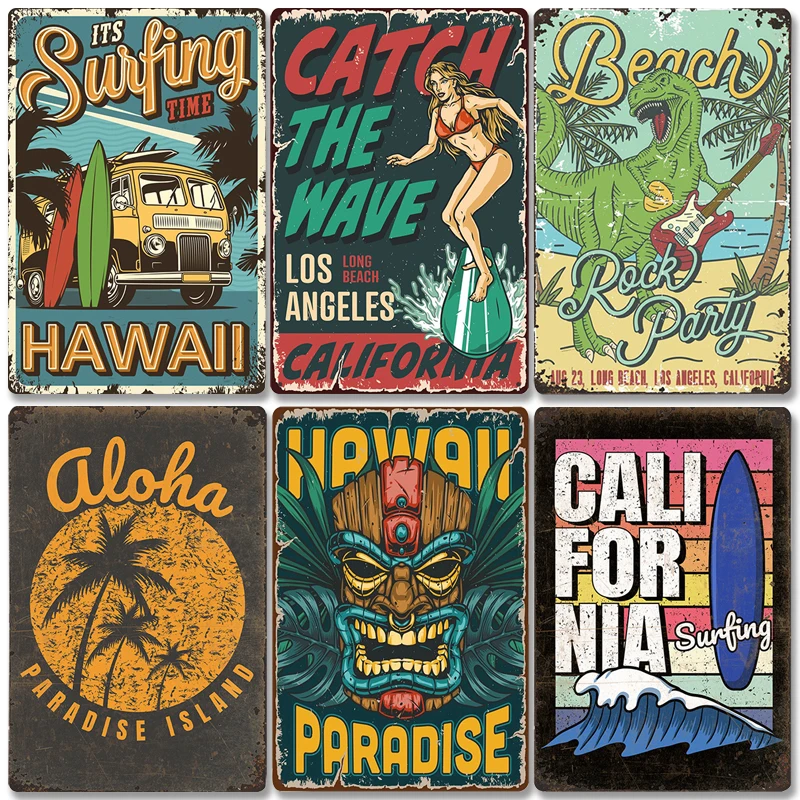The image depicts six vintage, weathered, vertical rectangular metal signs, each with unique designs and beach-themed graphics, grouped in two rows of three. The top left sign features a VW van with red and green surfboards leaning against it. In quirky text, it reads "It's Surfing Time" at the top, with "Hawaii" at the bottom, silhouetted palm trees in the background. The top middle sign reads "Catch the Wave, Los Angeles, Long Beach, California," showcasing a woman in a red bikini surfing on a green surfboard amidst waves. The top right sign is playful, displaying a green Tyrannosaurus Rex playing a red guitar, with palm trees and ocean water in the background. It reads "Beach" in yellow cursive at the top, with "Rock Party" in blue and red text and "August 23, Long Beach, Los Angeles, California" at the bottom. On the bottom left, the sign reads "Aloha, Paradise Island," featuring a large yellow circle with silhouetted palm trees inside. The bottom middle sign showcases a tiki mask with gold rings around its eyes, blue metallic lips, and eyebrows, and palm tree leaves extending from the sides. It reads "Hawaii Paradise" in yellow text above and below the mask. The bottom right sign has horizontal lines in colors resembling a sunset, with "California" written in large white text and a blue surfboard with "Surfing" in white cursive. At the bottom is a simple illustration of a blue and white wave.